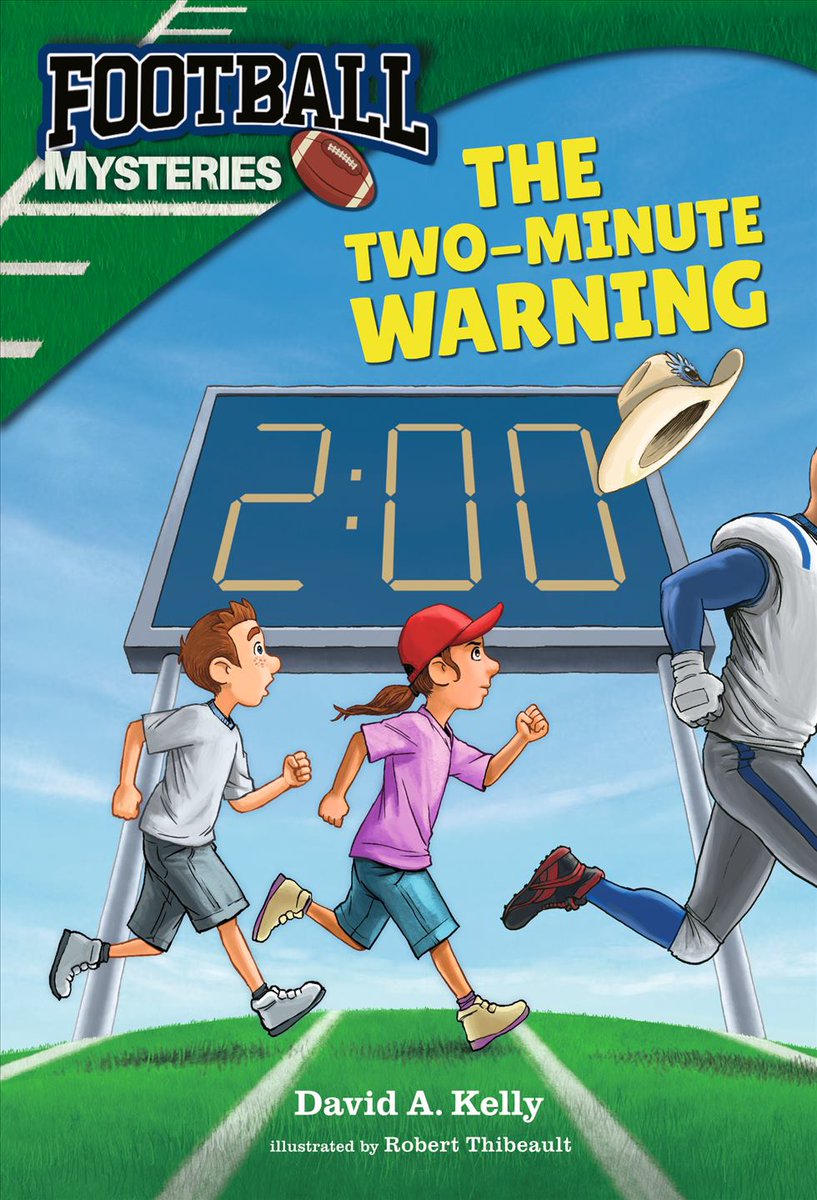The cover of the book titled "The Two Minute Warning," part of the "Football Mysteries" series, vividly captures a dynamic scene on a football field. In the forefront, a football player wearing a gray, blue, and white uniform dashes across the field, with red cleats on his feet, gloves on his hands, and a cowboy hat flying off behind him. His face is not visible. Trailing him, a girl in a pink shirt, denim shorts, and a red cap races ahead of a boy dressed in a gray shirt, gray pants, and gray shoes. The scoreboard in the background displays "2:00" in a digital format, indicating two minutes left. Above this engaging illustration, the book’s title "The Two Minute Warning" is prominently featured in yellow letters, with the series name "Football Mysteries" and a football graphic at the top. The sky is visible through an opening with clouds and a blue hue. At the bottom of the cover, it reads: "David A. Kelly, illustrated by Robert Theiboldt."